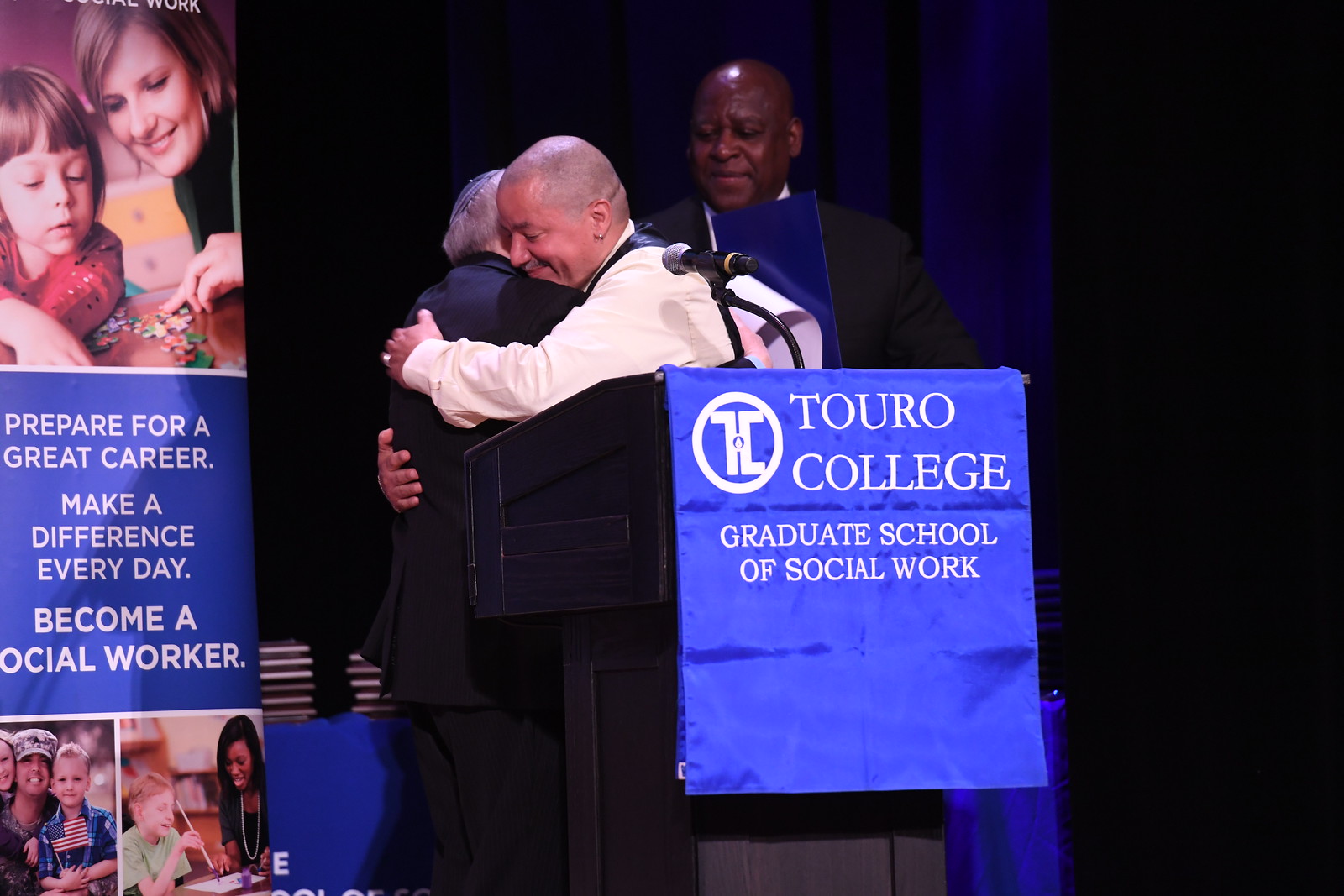The image features a touching moment on a stage with a black background, where two Caucasian men are embracing in front of a podium. The man on the right is bald, wearing a white tuxedo shirt paired with a black vest, and has an earring in his left ear. He is hugging another man in a black suit who has a Jewish cap on the back of his head. Behind them, a man in a black robe is observing the scene, holding what appears to be a diploma. The podium is draped with a blue banner that reads "Touro College Graduate School of Social Work" and includes an insignia on the left. To the left of the podium, there is a poster featuring a series of images: at the top, a mother and a child smiling while working on a puzzle, captioned "Prepare for a great career. Make a difference every day. Become a social worker." Below this, there's a picture of a service member with his wife and son holding an American flag, and at the bottom, a woman teaching a young child how to paint.